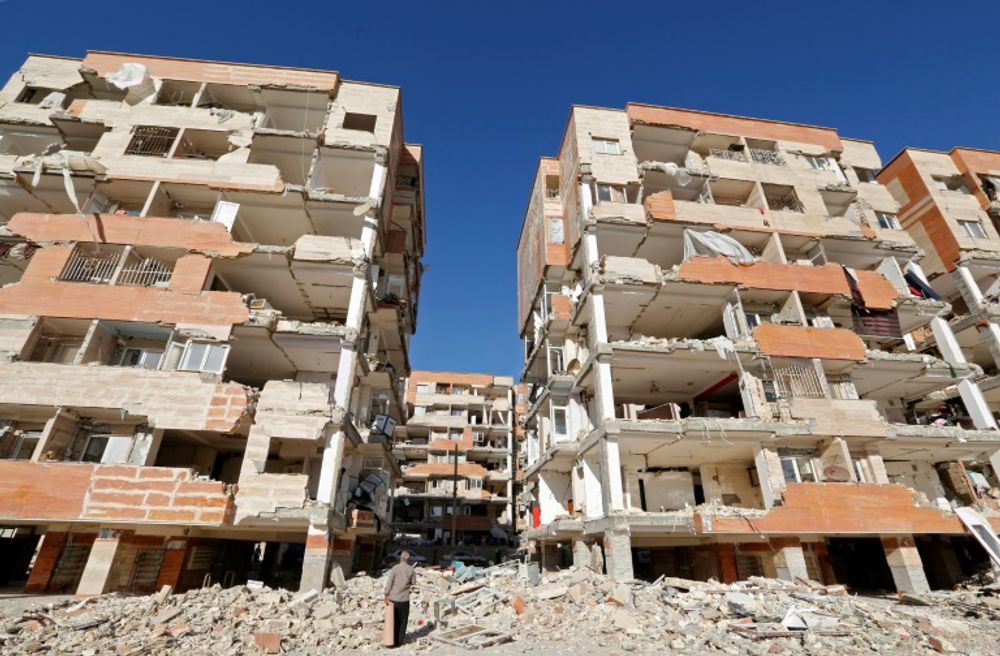In the photograph, an impossibly clear, beautiful blue sky starkly contrasts with the grim scene below. The image, taken from a low vantage point, captures a war-torn area with bombed-out apartment buildings standing about six or seven stories high. These buildings, likely located in Gaza or possibly Eastern Europe, are predominantly made of light sandy-colored concrete with remnants of a terracotta-colored brick facade, which once added decorative elements before the bombardment. The heavily damaged structures reveal white interiors through half-collapsed walls and crumbling bricks, indicating the severe extent of the destruction. In the immediate foreground, a large pile of rubble dominates the scene, stretching across the bottom of the image. Amidst the debris, a man in a gray coat or sweater stands on the rubble, seemingly looking up at the devastation around him, trying to make sense of the chaos. While the exact origin of the attack is unclear, the uniformity of the buildings and the extensive damage depicted paint a harrowing picture of conflict and ruin.